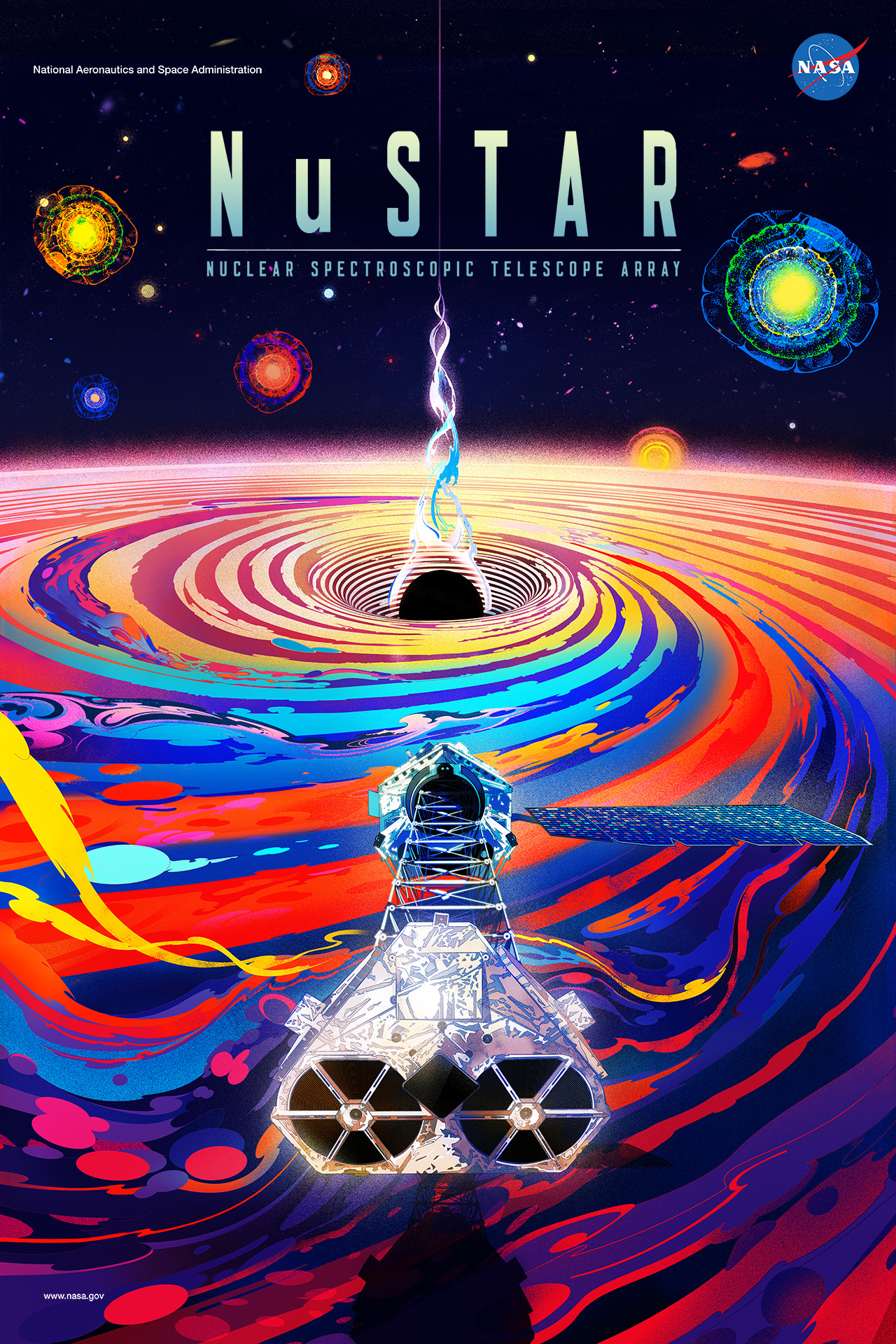The poster is an illustration for the NASA NuSTAR (Nuclear Spectroscopic Telescope Array) mission. In the upper right-hand corner, there's a prominent NASA logo, a blue circle with white lettering and a red streak. The central image depicts a vibrant, artistically rendered planet with a twisting black sphere emerging from its surface, creating colorful spirals in hues of red, blue, purple, and yellow that expand outward like a whirlpool. Surrounding the planet, variously sized and colored stars populate the dark blue background. A satellite array is seen orbiting this planet, positioned over the swirling, multicolored spirals. At the top left, "National Aeronautics and Space Administration" is inscribed in white font, further emphasizing the poster's connection to NASA. The overall aesthetic is both scientific and whimsical, blending elements of space and art to convey the complexities of the NuSTAR mission.